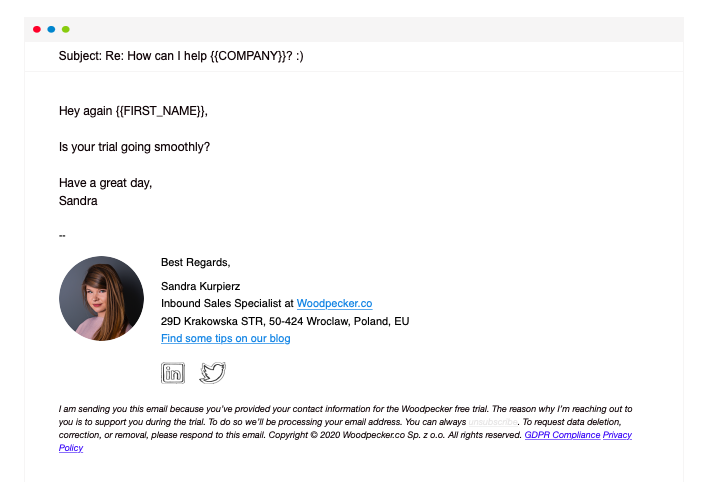This screenshot captures an email from Woodpecker.co. At the top, there's a light gray bar featuring three small circles: a red circle, a blue circle, and a green circle, positioned on the left. Below the bar, the subject line reads "RE: How Can I Help?" followed by "[[Company]]".

The email begins with a salutation, "Hey again, [[first_name]],". The body of the email inquires, "Is your trial going smoothly?" and concludes with a friendly note, "Have a great day," signed "Sandra." Accompanying Sandra's sign-off is a round profile picture of a woman with long light brown hair.

To the right of the profile picture, the sender's details read:
"Best regards,
Sandra [Unpronounceable Last Name]
Inbound Sales Specialist at Woodpecker.co
29 D Krakowska STR
50-424 Wrocław, Poland, EU"

Beneath Sandra’s contact information, there's a suggestion to "Find some tips on our blog" followed by the Twitter bird icon. 

A footer notice states: "I'm sending you this email because you provided your contact information for the Woodpecker free trial. The reason why I'm reaching out to you is to support you during your trial. To do so, we'll be processing your email address. You can always [contact us] to request data deletion, correction, or removal. Please respond to this email if you have any questions."

The email concludes with a copyright notice: "© Woodpecker.co".